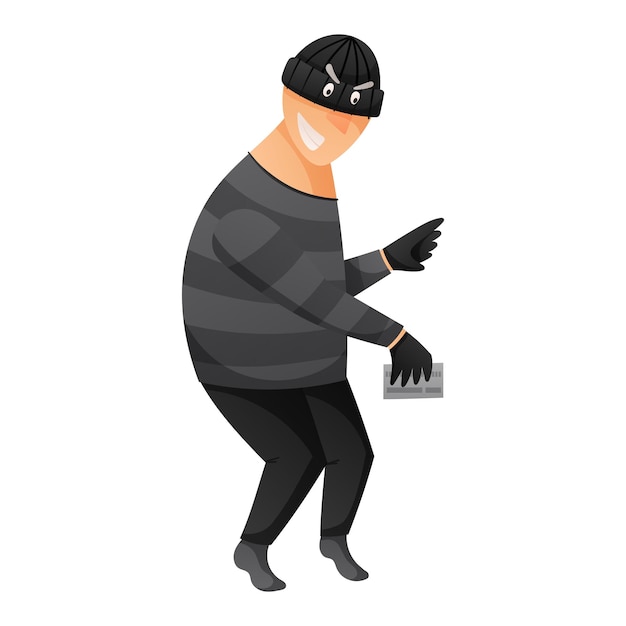The image is a computer-generated cartoon of a burglar, depicted with a distinctive mix of gray and black attire. The character wears a dark gray and light gray striped long-sleeved sweater, black pants, and black gloves. His footwear consists of gray socks. A notable feature is his black beanie, which covers his head but humorously includes eye and eyebrow details printed on it, giving the illusion that his eyes and eyebrows are on the hat itself. His face, showing a flesh-toned nose and a wide, cheeky smile, adds to the playful nature of the image. In his right hand, he holds a small rectangular white card, possibly a key card, and he appears to be tiptoeing, further emphasizing his burglar persona. The background is a stark white, keeping the focus solely on the animated thief.